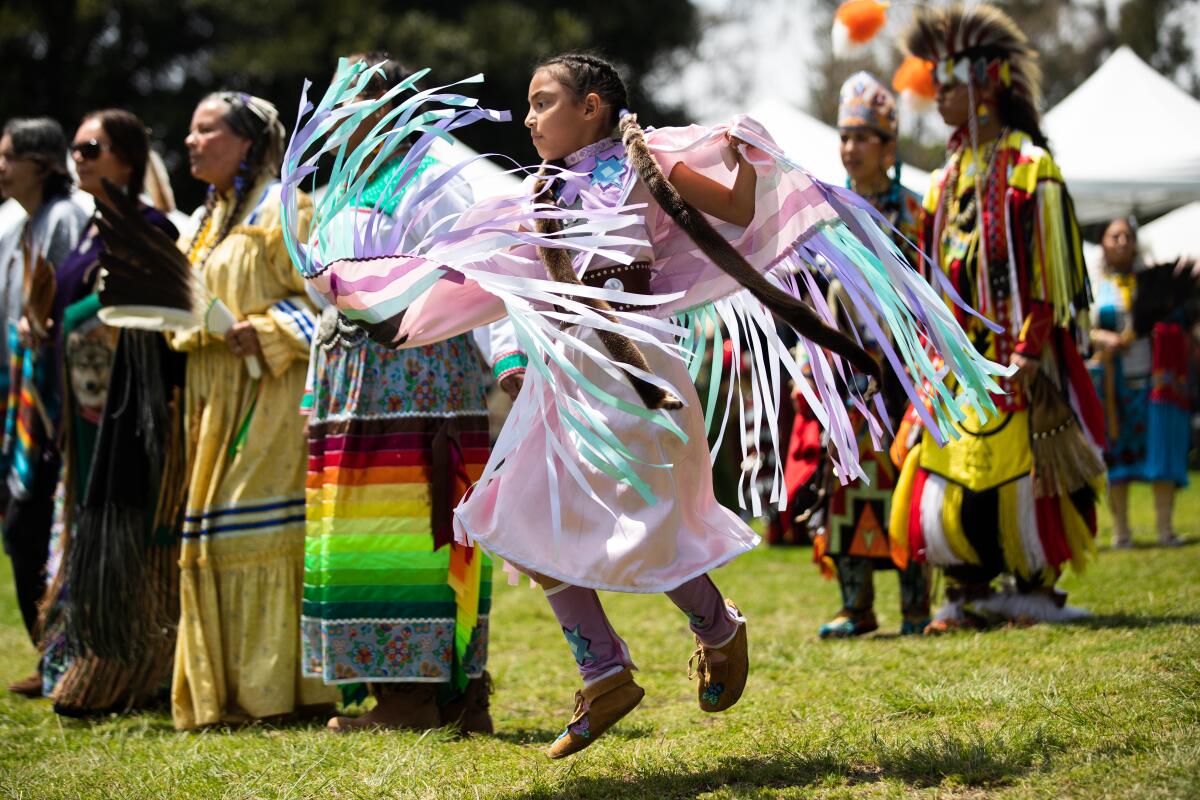In this vibrant and dynamic color photograph, we see a lively scene at a traditional American Indian festival, set outdoors under a bright, sunny sky. The centerpiece of the image is a young Native American girl, estimated to be between 10 to 13 years old. She is captivatingly twirling in the middle of the photograph, donning a knee-length pink robe adorned with sashes and a matching cape. The cape features long, flowing fringes in green, white, aqua, and purple, some of which she holds in her hands as she spins with joyful energy. Her hair is styled in long pigtails, and she wears traditional moccasins on her feet.

Surrounding her are numerous participants clad in customary colorful outfits, contributing to the festive atmosphere. To her right, a man stands out in a feathered headdress and a knee-length outfit that blends yellow, red, and white. To her left, amidst a throng of festival-goers, is a woman presumed to be wearing a multicolored dress in shades of red, yellow, and green, while another figure next to her is dressed entirely in yellow. Further left, a person in black with sunglasses and another individual are visible. The participants appear to be engaged in some sort of ritual or parade, possibly a springtime celebration.

The background features white canopy tents to the right and a serene grove of trees, with people milling about and enjoying the festivities on the grass. The vivid display of traditional attire, the excitement of the young dancer, and the overall ambiance of cultural celebration are beautifully captured in the frame.